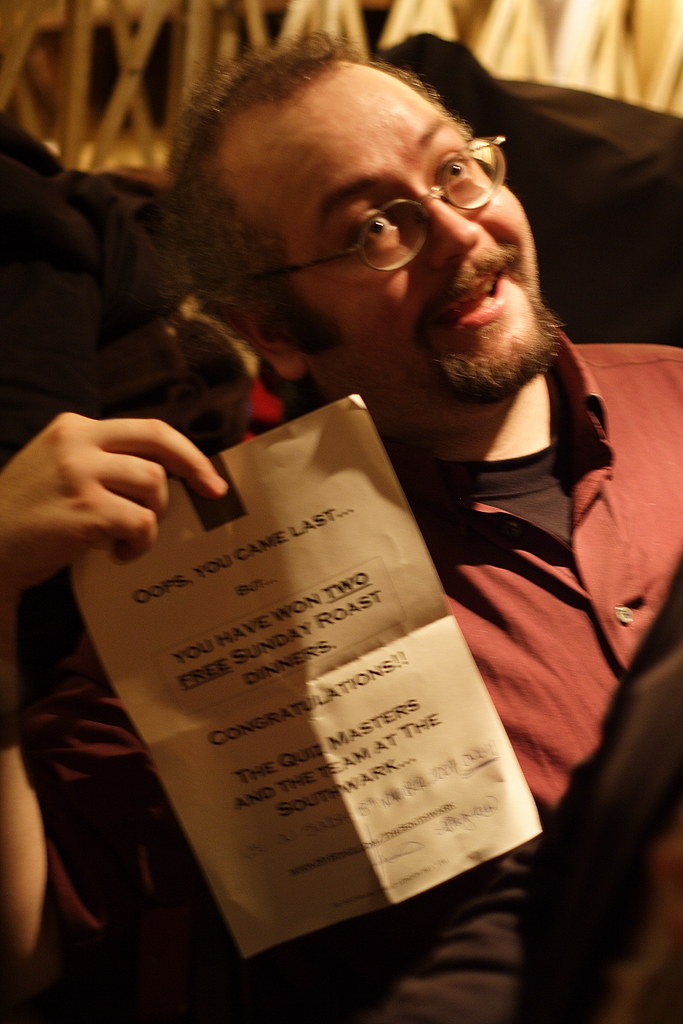This indoor nighttime photo captures a thrilled gentleman with round glasses, a full beard, and a goatee, prominently smiling with his head slightly tilted to the right. He is dressed in a maroon collared shirt over a black t-shirt. His mouth is open in a joyful expression, with his eyes wide open, looking to the right of the camera. The warm glow of overhead lights illuminates his face, adding to the lively atmosphere. Holding the paper from the top with his right hand, he proudly displays a sheet that reads, "Oops, you came last, but you have won two free Sunday roast dinners. Congratulations from the Quizmasters and the team at South Ork." The photo features a dark background with indistinct elements, focusing on the jubilant man. Handwritten, illegible phrases are also visible on the paper.